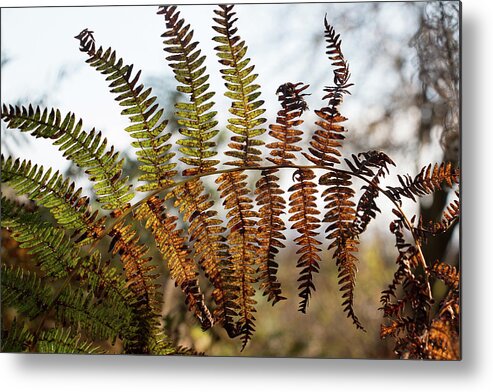This photograph captures an intricate portrait of a fern leaf prominently set against a blurred outdoor background. The main feature is a large fern branch that elegantly arches from the right side of the frame to the left, with its peak roughly centered. The fern fronds exhibit a visual gradient of vitality: the upper fronds are predominantly green, some tinged with brown, and the lower fronds show signs of aging or sun damage, appearing brown and shriveled. This scene suggests a mid-season transition, possibly autumn, as the mixed foliage behind the fern appears light green while the sky above is a very light blue, hinting at a clear, daylight setting. The background is filled with indistinguishable but evidently lush greenery, emphasizing the isolation and detailed clarity of the fern branch in focus. The overall atmosphere conveyed is one of natural beauty amidst the cycles of life and decay, giving it a slightly melancholic, yet serene feel.